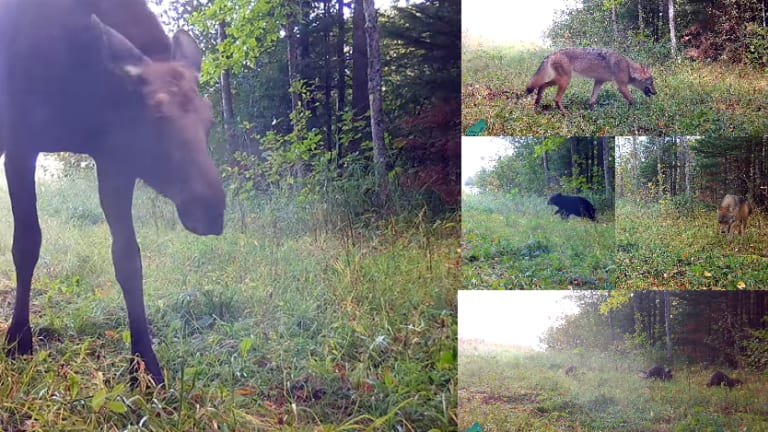The image is a composite of five individual pictures showcasing various animals in their natural habitats. The most prominent picture on the left side features a large, dark brown moose without antlers, walking through an area of tall grass and surrounded by trees. To the right of the moose, there are four smaller pictures arranged vertically. The top picture depicts a coyote walking through a grass-covered area. Beneath it, a brown bear is shown in a similar grassy setting. Adjacent to the bear, there is another coyote, this time facing forward. The bottom picture captures two small bear cubs, also amidst the greenery of the forest. Each animal appears to be looking down, possibly searching for food, and the entire scene is immersed in the wilderness with no other objects or text present.